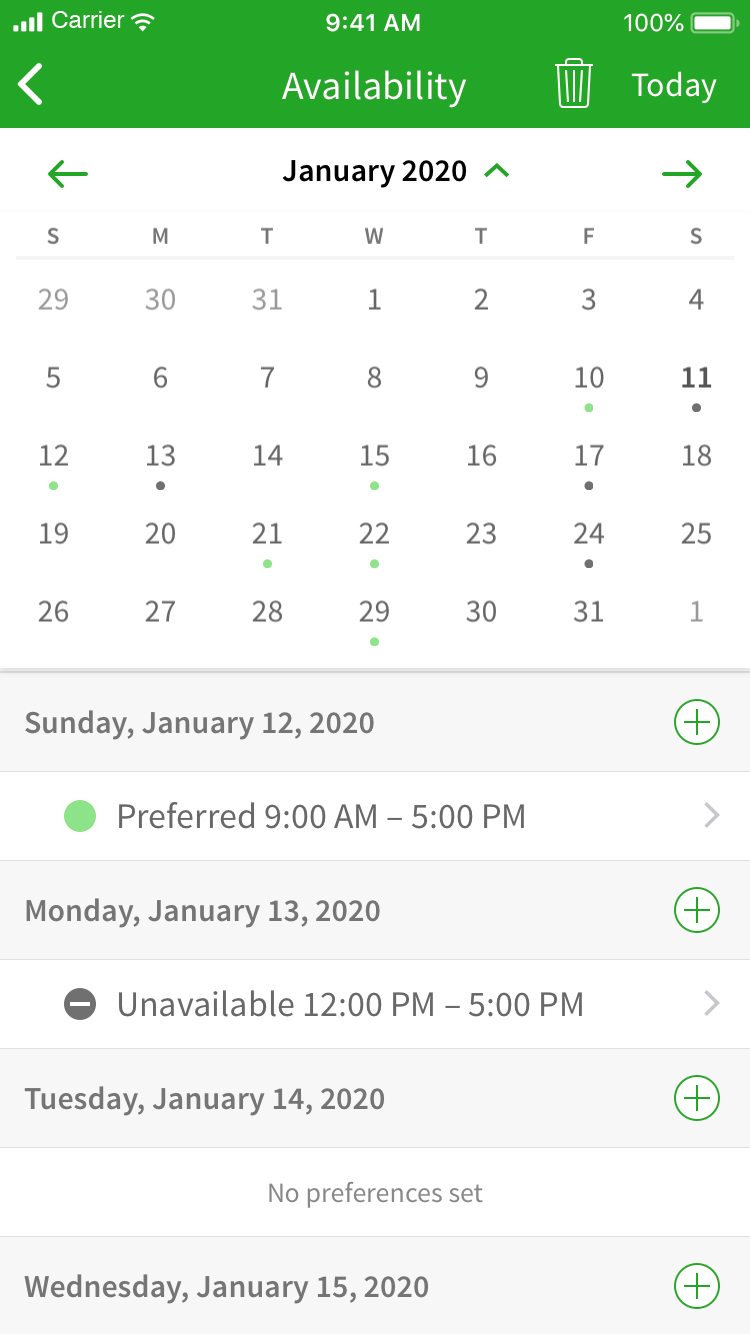The image displays a smartphone screen with a calendar app open, showcasing the user's availability. The calendar is set against a green header at the top, with the word "Availability" prominently written in white letters. Adjacent to this title, there is a white trash can icon and a label indicating "Today." The phone's status bar reveals a fully charged battery at 100%, the current time as 9:41 AM, WiFi connectivity with full signal strength, and a five-bar phone signal.

The calendar covers the month of January 2020, beginning from December 29, 2019, and extending to February 1, 2020. The days are organized in a traditional Sunday to Saturday format. Specific dates and times for availability are noted: On Sunday, January 12th, 2020, the user is marked as preferred from 9 AM to 5 PM. On Monday, January 13th, 2020, the user is unavailable from 12 PM to 5 PM. Both Tuesday, January 14th, and Wednesday, January 15th, 2020, are listed without any preference settings. 

Next to these dates, white circles with green plus signs and green borders indicate areas where additional settings or notes can be added. An arrow next to the availability times implies options for editing or modifying existing entries.